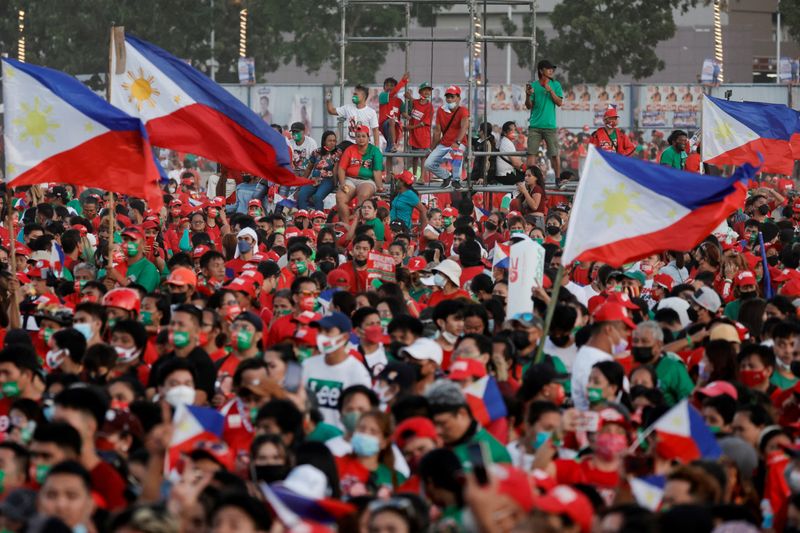This image captures a dynamic scene of what appears to be a large protest or rally in the Philippines. The crowd, extending to the horizon, predominantly consists of people wearing green and red clothing, with many sporting masks in red, green, or white. Filipino flags, characterized by their blue, red, and white design with a yellow sun on a white triangle, are prominently displayed throughout the crowd, contrasting the colors worn by the protestors.

The energy in the image feels intense and charged, suggesting a significant degree of unrest or passionate advocacy. A tall, metallic scaffold or stanchion towards the center of the image holds several individuals, including a man in a gray or green shirt and tan shorts, who overlook the crowd from their elevated position. These people, along with most of the crowd, generally face the same direction, as if focusing on a central point of interest or speaker outside the frame.

In the background, a white wall adorned with posters stands behind a line of trees, providing a backdrop to the scene. The overall atmosphere, coupled with the visual elements, implies a large-scale public gathering with significant social or political implications.